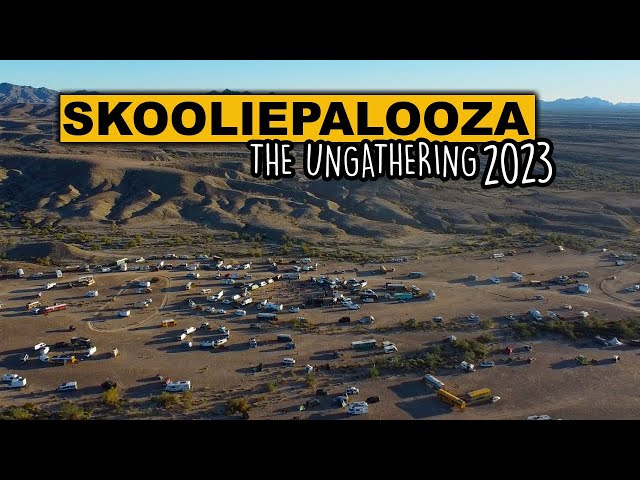The image captures an expansive aerial view of a vast, desert landscape scattered with numerous vehicles, primarily RVs and trucks, parked randomly across a wide, dry area. The background features brown, arid hills that accentuate the rural, mountainous terrain. It appears to be a large camping or gathering event named "Skooliepalooza The Ungathering 2023", hinted by the text prominently displayed on the image. "Skooliepalooza" is written in bold black font inside a yellow rectangular box at the top of the image, with "The Ungathering 2023" in white font bordered in black directly beneath it. Some dark green bushes sporadically dot the otherwise barren landscape, adding slight contrast to the scene. Despite the distant vantage point, the cluttered arrangement of the vehicles against the dry, grayish ground creates a striking visual emphasizing the scale and isolation of the event.